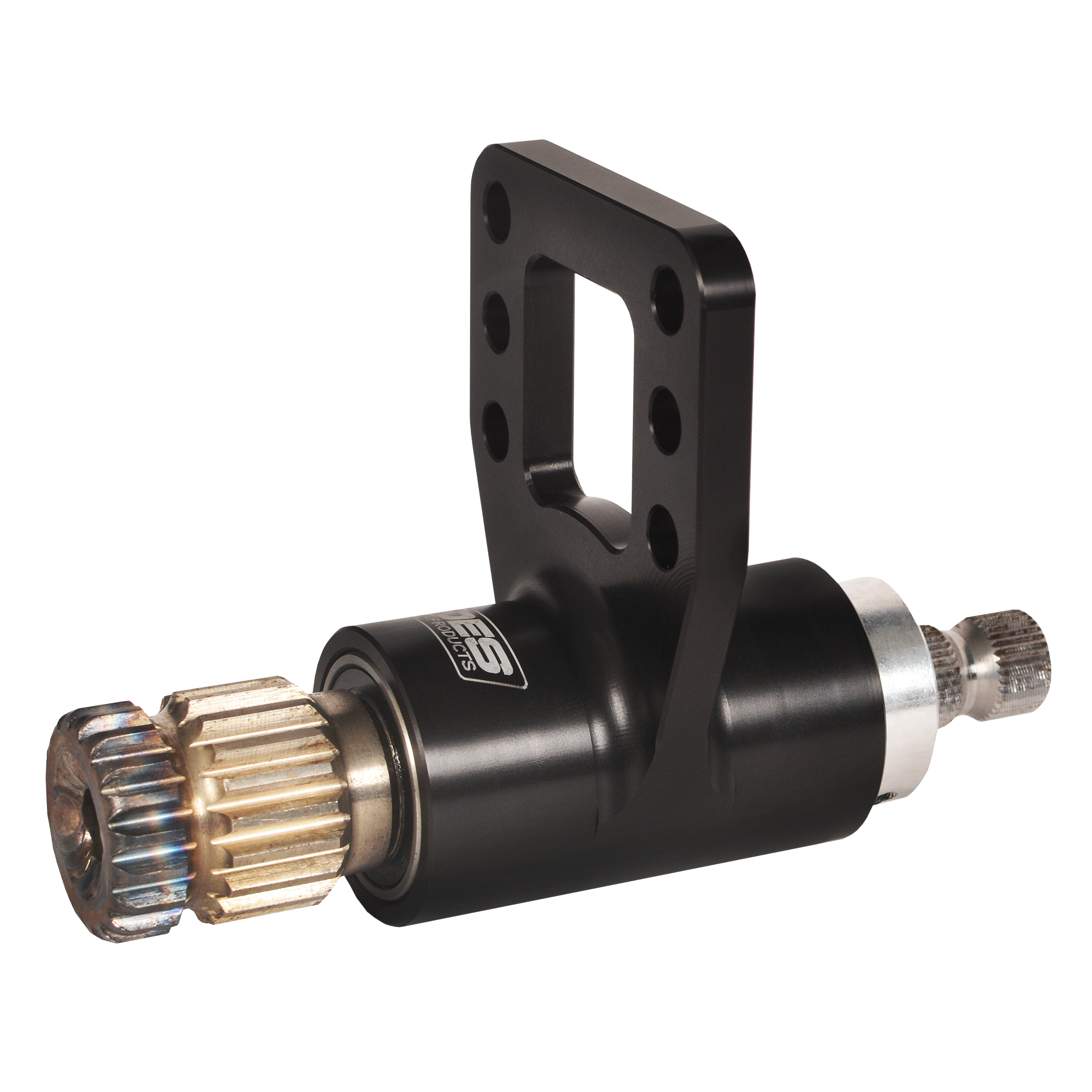This image showcases a complex machine set against a completely white background. On the left side of the machine, there are two prominent gears: one dark gray and one golden. Adjacent to these gears is a cylindrical body that is black in color. A label marked with "ES" and the word "products" is visible on this cylinder, which also features a black handle. The handle has a unique design, with a square-shaped cutout in the middle and circular cuts on either side. To the right of the cylindrical body are two silver gears, one of which shines with blue and red highlights. Additionally, a metallic piece resembling a narrow, unribbed faucet end extends further to the right. This intricate arrangement of parts creates a detailed and robust mechanical tool.